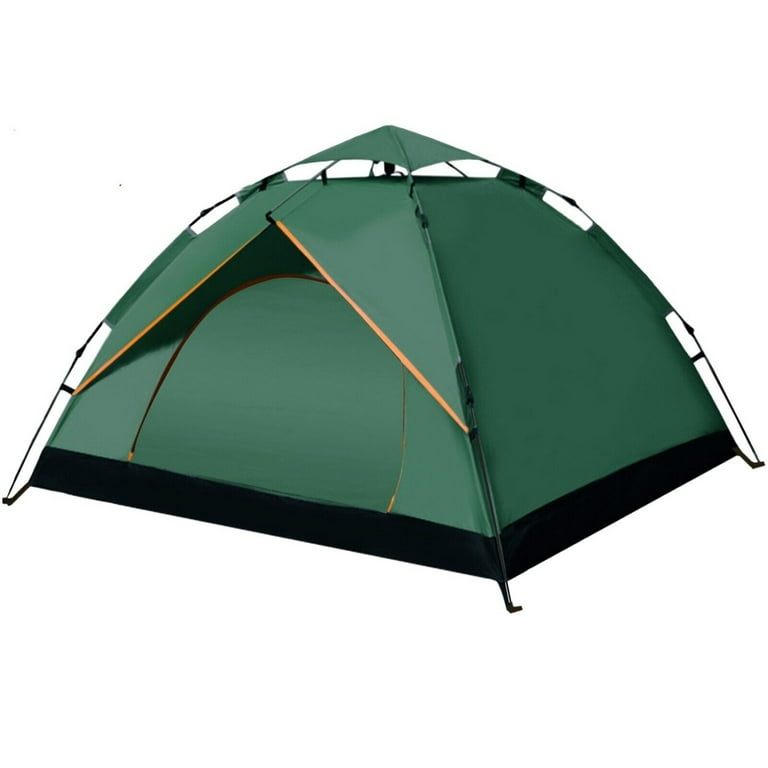This computer-generated, clip art-style drawing depicts a small, forest green tent set against a white background. The tent features four corners, with a design that tapers into rounded triangular shapes, giving it a somewhat pointy top that curves outwards at the sides. The front of the tent, situated slightly to the left, has an orange border around an oval-shaped flap, which serves as the entrance. Above this oval opening, there are two small triangular green pieces, with a dark black spot to the top left, possibly indicating another opening or vent.

The tent is supported by thin black rods, likely made of metal or plastic, that curve upwards and converge at the center, ensuring the structure's stability. These rods are affixed to the ground, demonstrating the tent's setup. The bottom edge of the tent is bordered by a black rectangular strip. On the right side, the green fabric wall remains plain and uninterrupted. The empty white background emphasizes the tent as the focal point, suggesting an outdoor setting despite the lack of contextual elements.